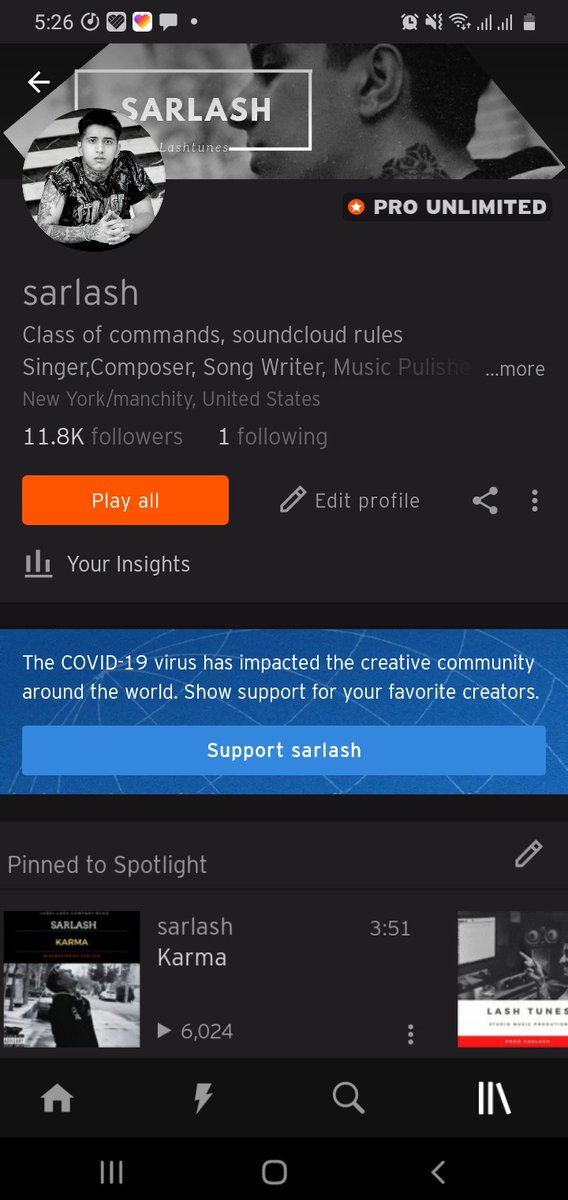The background of the image is dark grey. In the upper part of the image, there is a partial view of a phone screen displaying the time "5:26" in white text. Below this, prominently featured, is a black-and-white side profile of a man looking towards the left. His face is above the text "S-A-R-L-A-S-H" which is written in white and framed by a white border. 

Next to this, there is a grey-scale profile picture of the same man, this time looking directly at the camera. He has a tattoo sleeve on his right arm and is possibly of Hispanic descent. His shirt color is indeterminate due to the monochrome presentation.

Below the images, the text "S-A-R-L-A-S-H" appears again, followed by detailed information: "Clash of Commands, SoundCloud rules, singer, composer, songwriter, music publisher," and an ellipsis indicating more. His location is listed as "New York/Manchester, United States" with "11.8K followers, one following."

An orange rectangular button labelled "Play It All" is visible, next to a pen icon and the words "Edit Profile." Below this is a section titled "Your Insights."

At the bottom, a blue rectangle contains a message in white text: "The COVID-19 virus has impacted the creative community around the world. Show support for your favorite creators." Another blue rectangle underneath reads "Support SART Latch."